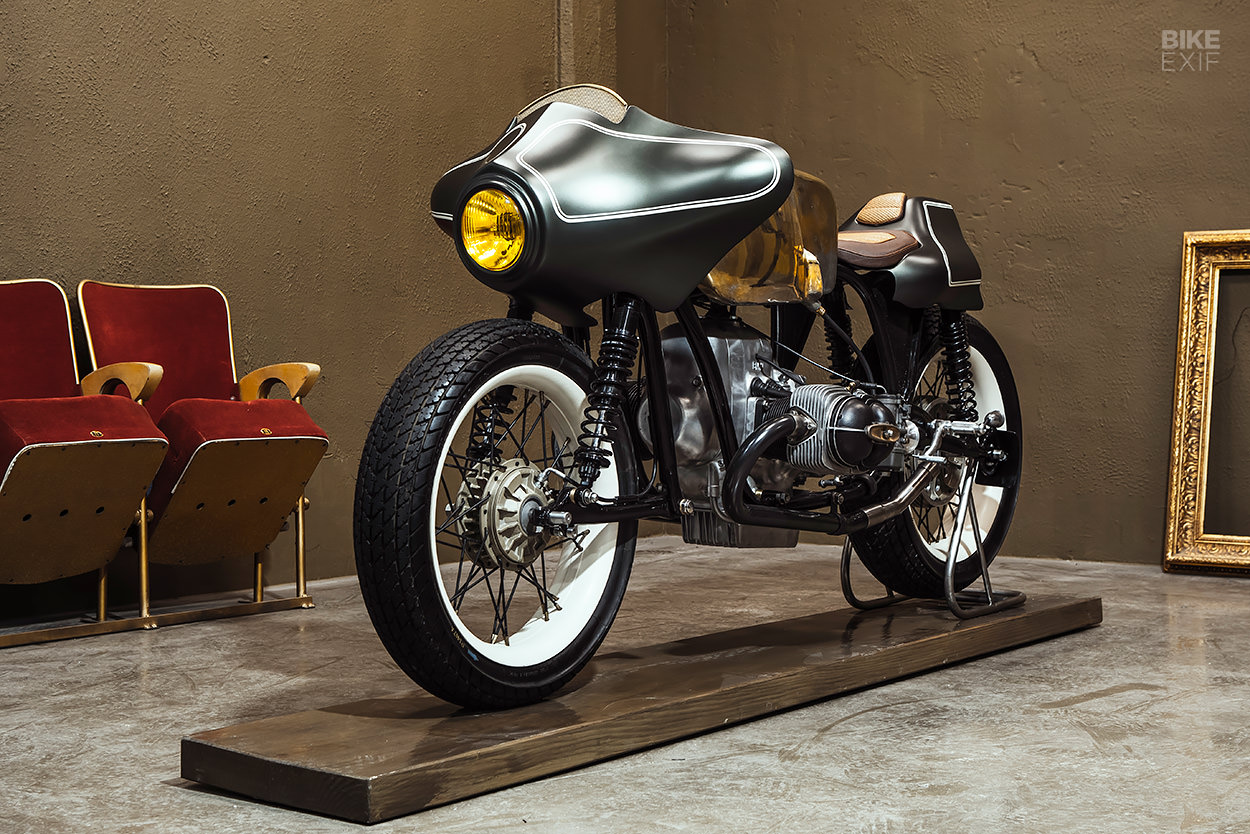The image features a sleek, black motorcycle with a futuristic design, prominently displayed on a small wooden stand. The motorcycle boasts a shiny matte black finish, with its machinery parts exposed in the center. Its front portion is equipped with one large, circular amber-colored headlight, positioned centrally with metal components above it. The front and rear of the motorcycle are fitted with spring shocks, and the seat is designed to be flat in the front while angling upwards at the back. 

The tires are thick and black, contrasting with the white wheels. The motorcycle is situated in a room with gray floors and brown walls. Two red velvet chairs with brown handles are positioned on the left side of the image, folded up. On the right side, a gold picture frame is visible in the background. The top right corner of the image features the text "bike EXIF" in bold white lettering, although this section appears somewhat faded.

The scene is detailed down to the mixed brown and white marks on the metal floor beneath the wooden stand, highlighting the careful presentation of the motorcycle.